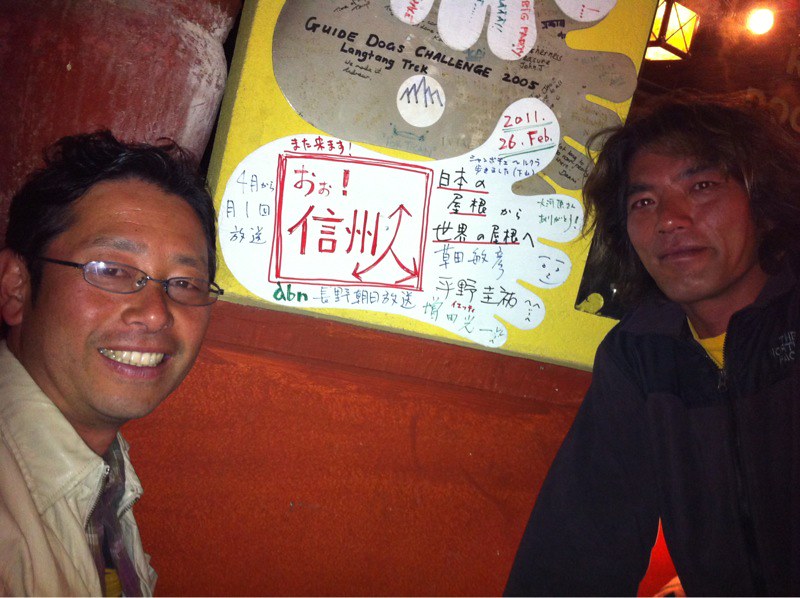The photograph captures two middle-aged men of Filipino or East Asian descent standing against a vibrant red wall. Despite the dim lighting, the man on the right is clearly visible from the chest up, wearing a black sweatshirt over a yellow shirt, and he has chin-length hair and a loose smile. The man on the left is adorned in a cream-colored (or light tan) jacket, possibly over a plaid shirt, and he sports glasses, short hair, and a vivid smile that reveals his teeth. 

Both men are looking directly at the camera, suggesting the photo might be a selfie or taken by someone else. Between them is an intriguingly angled poster with a bright yellow background featuring text and symbols in what appears to be Japanese or Chinese. The poster prominently displays the text "Guide Dogs Challenge 2005, Long Tang Trek" along with artistic depictions of white and gray feet and several colored drawings of mountains amidst red, blue, and black text.